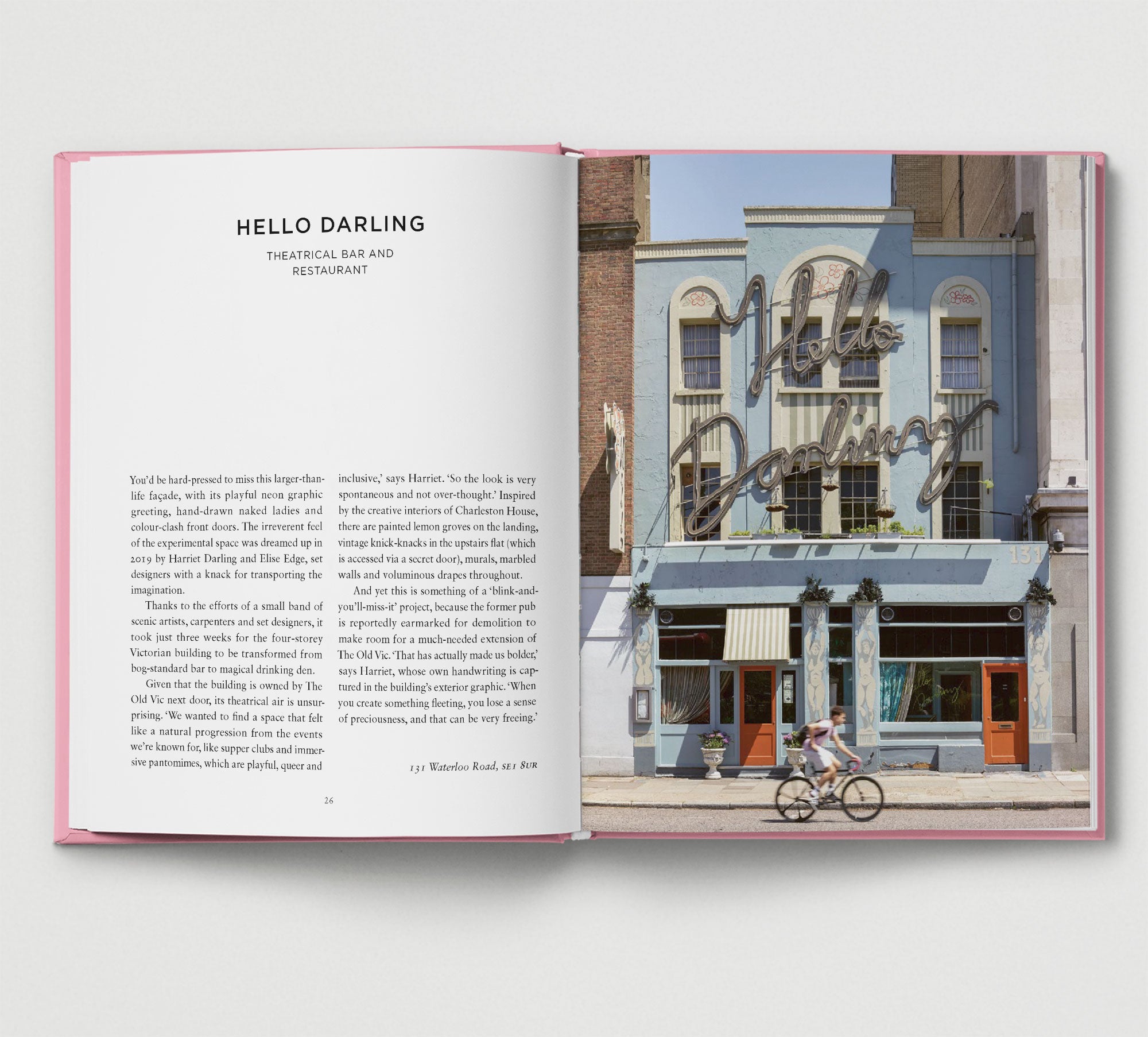The image depicts an open book with pink edges, laying on a light gray surface, revealing page 26. On the left page, in large, bold black letters at the top center, it reads "Hello Darling." Below this, it says "Theatrical Barn Restaurant" in smaller print. Further down, the page is mostly blank, with two columns of text at the bottom half consisting of several paragraphs, which likely describe the restaurant. Additionally, there is an address, "131 Waterloo Road," at the bottom. The right page features a large daytime photograph of the restaurant’s exterior, a light blue, three-story building with orange doors and planters in front. The building has a decorative sign reading "Hello Darling" in cursive, which spans diagonally across the top two floors. The photo also captures a man biking to the right on the street in front of the building, and there are some hanging plants above the first story, contributing to the quaint urban scene.